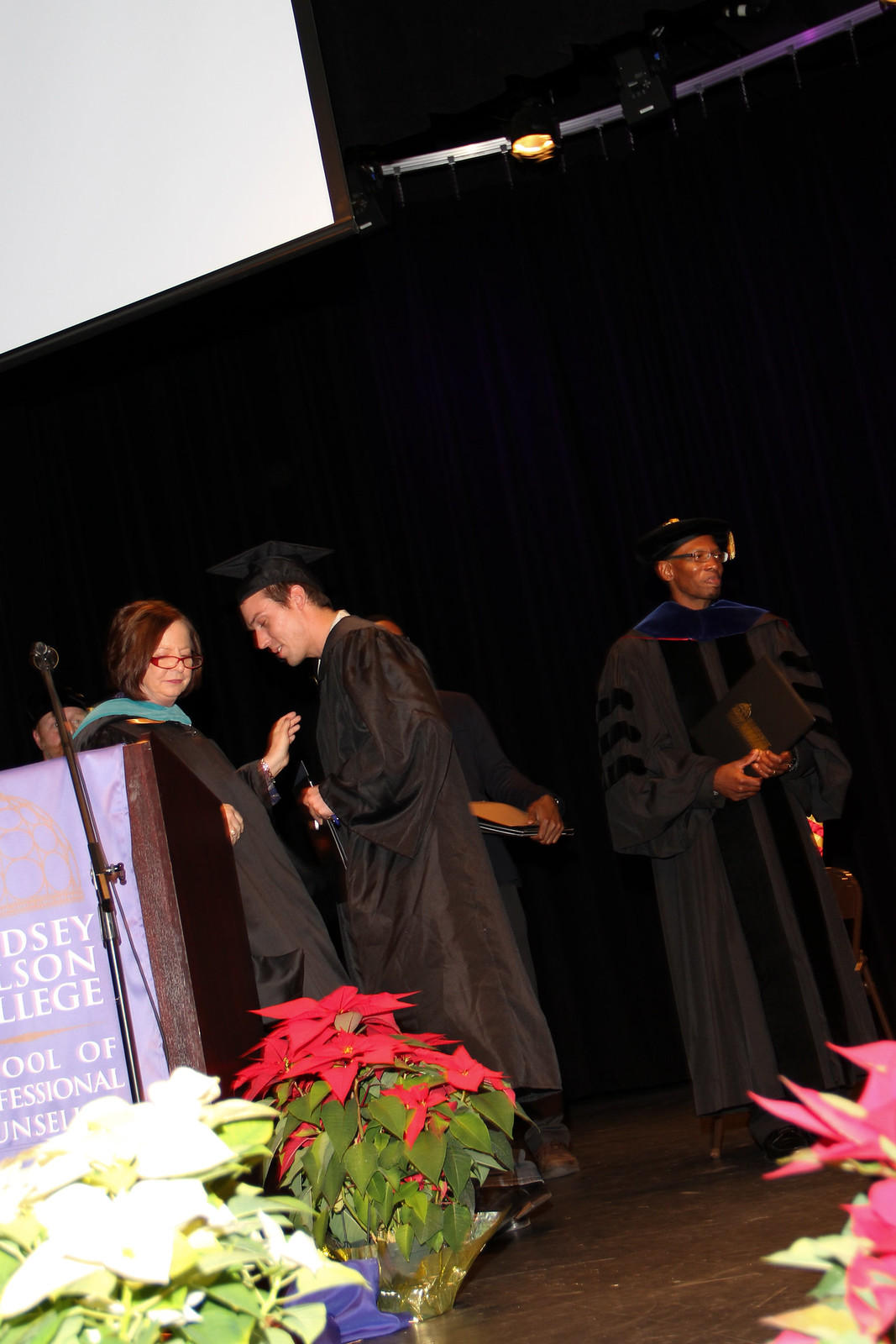This vibrant color photograph captures a graduation ceremony held indoors in an auditorium. On stage, five individuals clad in black caps and gowns signify the solemnity of the occasion. To the left, a podium draped with a light purple banner featuring white writing reads "D.S.E. S.O.N. College School of Professional Counseling." Beside the podium stands a woman with a turquoise scarf and red glasses, seemingly poised to hand a diploma to a young male graduate. Next to him is another man, distinguished by his black graduation gown and cap adorned with a gold tassel, likely one of the speakers. The background is a simple black curtain, enhancing the focus on the ceremony's key participants. The stage's front is adorned with an array of poinsettias in white, red, and pink, adding a festive touch to the celebratory setting.